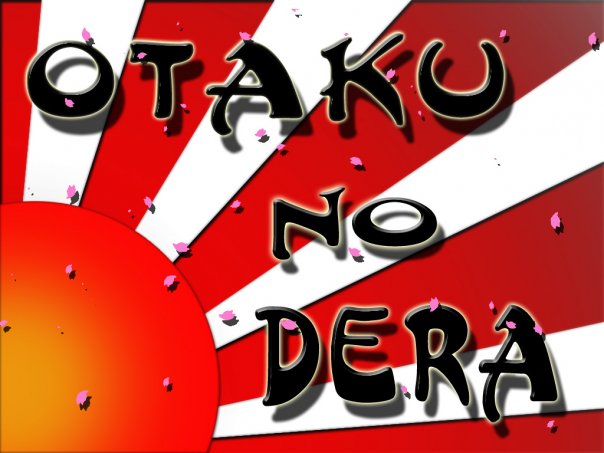The horizontal illustration features a striking design reminiscent of the rising sun from the Japanese flag. Dominating the lower left-hand corner is a partial orange disk with a hint of yellow at its center, interspersed with pink specks. Radiating from this disk are five thick, alternating rays in shades of red and white, each outlined by a thin black line on the left side against a vibrant red background. These rays fan out dramatically from the sun-like image. Superimposed over the entire composition are three bold lines of text in a black, stylized font with white outlines, reading "O-T-A-K-U" on the first line, "N-O" on the second, and "D-E-R-A" on the third. The text, along with the spread of pink specks resembling confetti, creates a dynamic and eye-catching focal point that enhances the overall graphic impact of the scene.